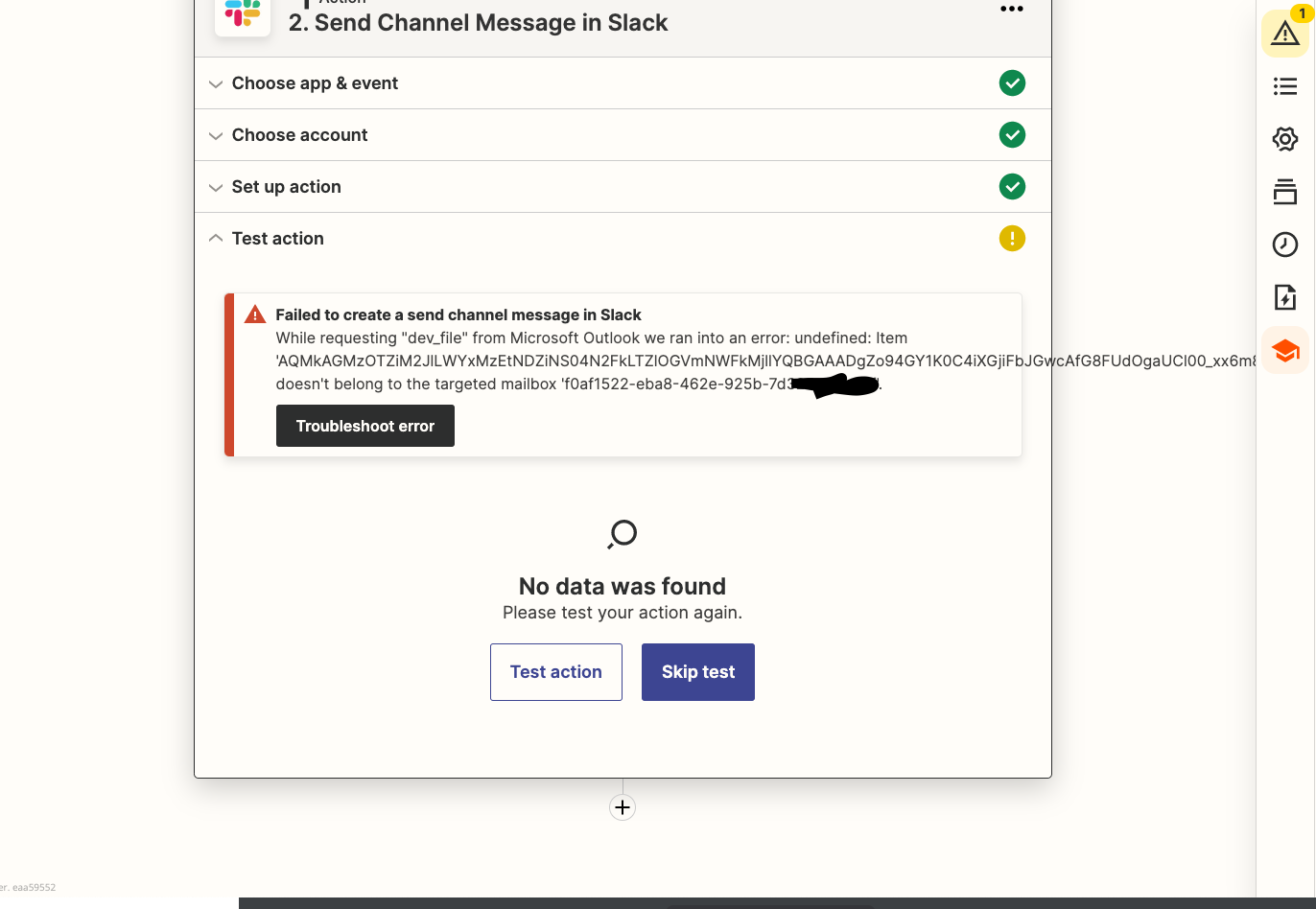The image displays a relatively square-shaped interface resembling a website or app window, aligned to the left and partially cut off at the top. At the top of this window is a multicolored logo made up of dots in teal, red, yellow, and green. To the right of the logo is the text "Send channel message in Slack" alongside three horizontal dots forming a menu.

Beneath this header are several horizontally separated sections. The first section features a down arrow followed by the text "Choose app and event," with a green checkmark indicating completion aligned to the right. The second section also contains a down arrow and reads "Choose account," accompanied by another green checkmark to the right. The third section follows the same layout, with a down arrow and the text "Set up action," and yet another green checkmark to the right.

The final section diverges slightly with an up arrow and the text "Test action," which is expanded and marked with a yellow exclamation point on the right, indicating a warning or issue. Additional text below this section seems to provide further context or instructions related to the warning.

Overall, the image appears to be part of a step-by-step setup process within a digital platform such as a task automation tool, indicating progress and errors at various stages.